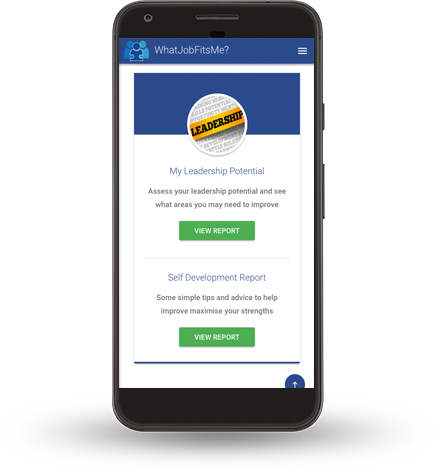The image displays a modern smartphone with a sleek black border. Notably, the device features a large button on the right side, likely for volume control, and a smaller button, presumably the power button. At the top of the phone, a thin, horizontal line serves as the speaker, and a tiny circle in the upper left corner houses the front camera. Additionally, the bottom of the phone is encased in a subtle black border.

On the phone's screen, an app is open, characterized by a blue header at the top. The header includes three blue icons resembling profile avatars alongside the text: "What Job Fits Me?". Below this are three horizontal white lines, suggesting a menu.

The main section of the app is set against a white background. Prominently displayed is a white circle accented by a gold strip, featuring the word "Leadership" in black letters. Below, the text "My Leadership Potential" introduces content encouraging users to assess their leadership skills and identify improvement areas. Two interactive options, "View Report" under "My Leadership Potential" and another "View Report" under "Self-Development Report" offer users a deeper dive into personal development tips and advice for maximizing strengths.